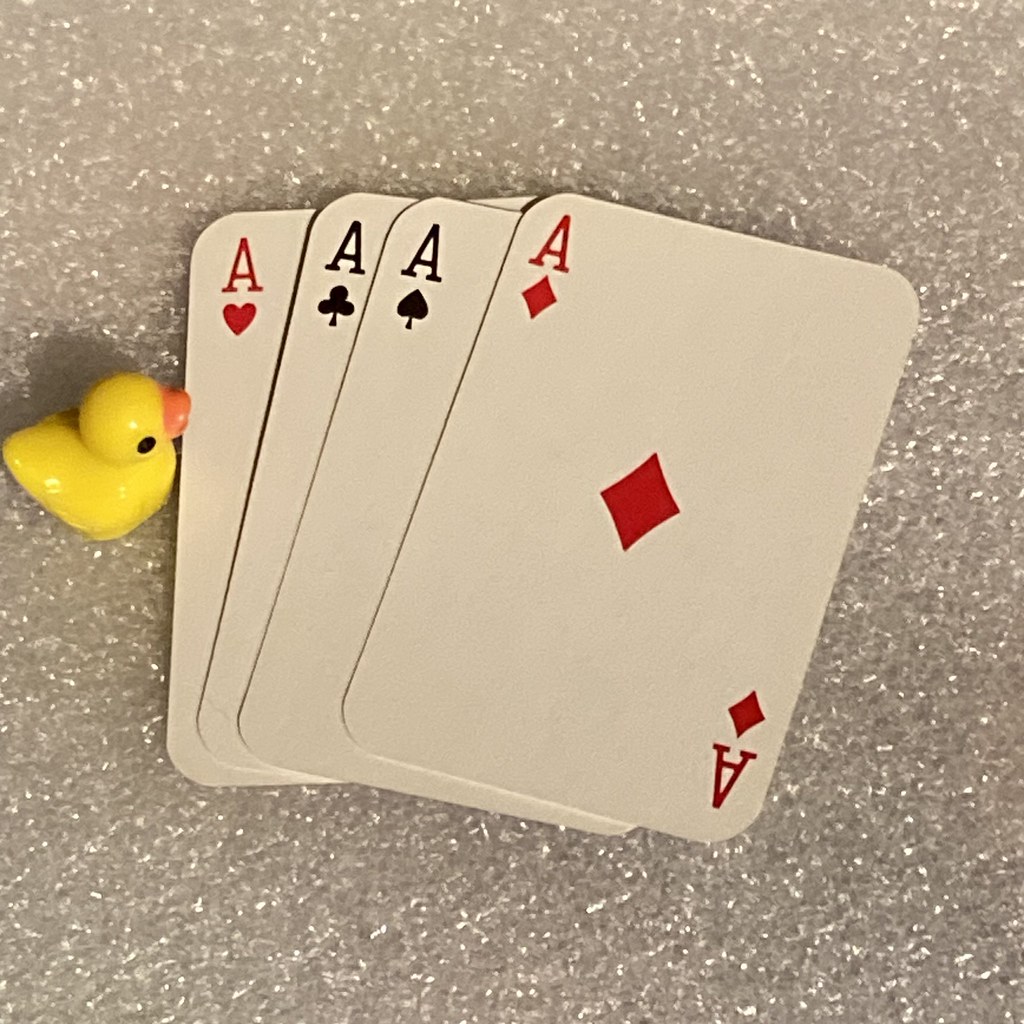The image features a fan arrangement of four playing cards, each with the white side facing up. At the forefront is the Ace of Diamonds, easily distinguished by its red diamond symbol positioned at the center and smaller diamond symbols at the top left and bottom right corners. Both corners also display capital "A" letters, with the card's design inverted at the bottom right.

Behind the Ace of Diamonds, three other aces are partially visible: the Ace of Spades in black, the Ace of Clubs in black, and another Ace of Diamonds in red, all fanned out to the left. 

Adjacent to the playing cards, on the right, is a small yellow rubber duck with one visible black eye and an orange bill. The duck's shiny, reflective surface suggests it could be made of either rubber or plastic. The perspective of the image captures the right side of the duck.

All of these items rest on a textured surface resembling charcoal-gray stone, with variations in shade likely caused by the play of light on its uneven surface. The stone texture is further detailed by sporadic white speckles.